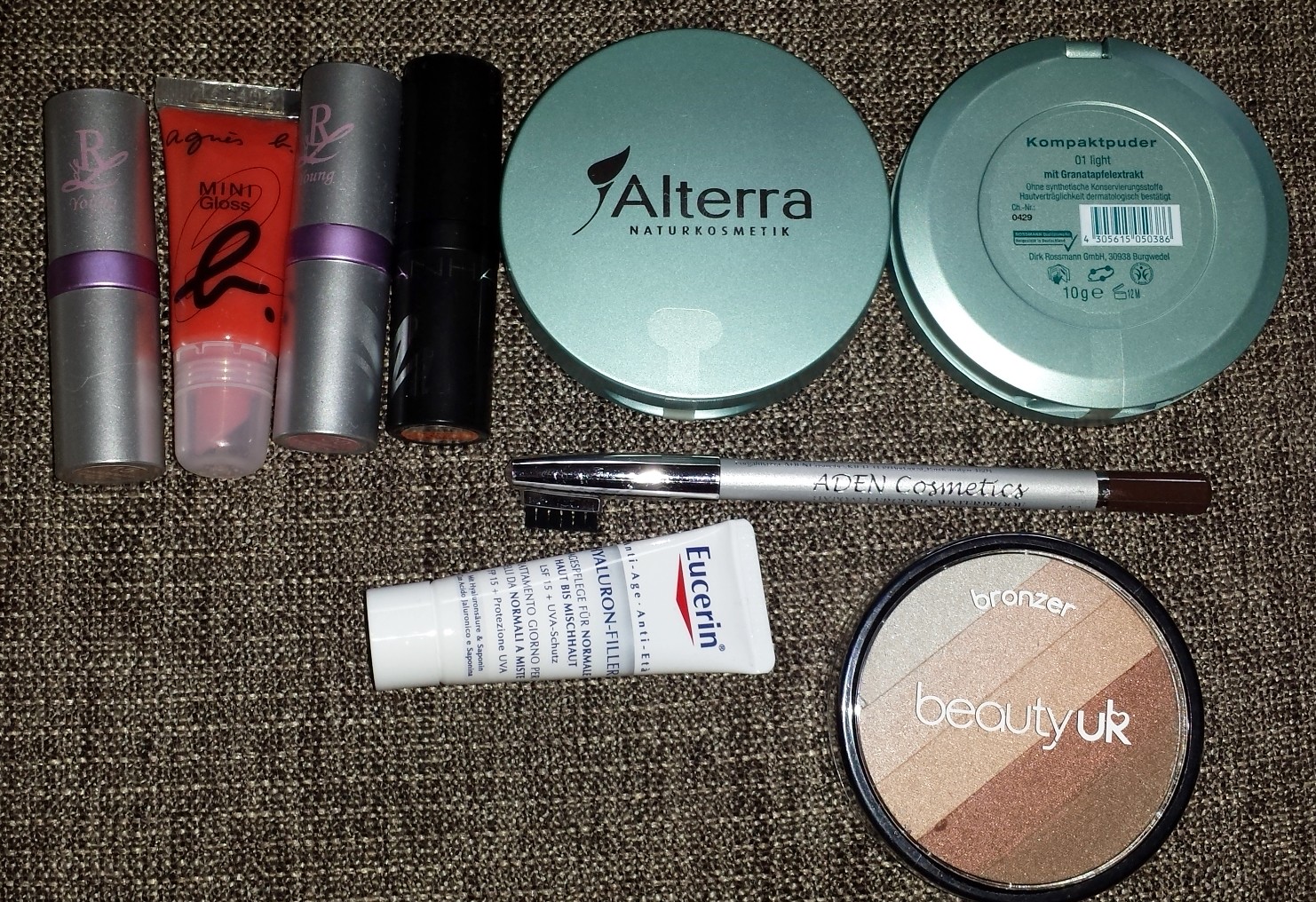The image is a detailed color photograph captured with a flash, oriented horizontally. The entire background is filled with a woven tweed-like fabric, setting a textured and cozy backdrop. At the top left corner, there is a neatly arranged row of lipsticks in various striking colors: red, silver, purple, and black. 

To the right of the lipsticks, there are two compact cases. The central compact is shown facing upwards, prominently displaying the brand name "Altera" on its cover. Next to it, the second compact is flipped upside down, revealing the text on its back.

A horizontally positioned color eye pencil, labeled "Aiden Cosmetics," divides the upper section of the image from the lower section. Below this pencil, there is a small tube of Eucerin lotion, identifiable by its distinctive packaging. Adjacent to the lotion, another compact case features a gradient of brown and pink shades, adding a subtle splash of color to the composition.

Overall, the photograph captures a meticulously organized array of makeup items, enhanced by a rich, woven background that adds depth and warmth to the scene.